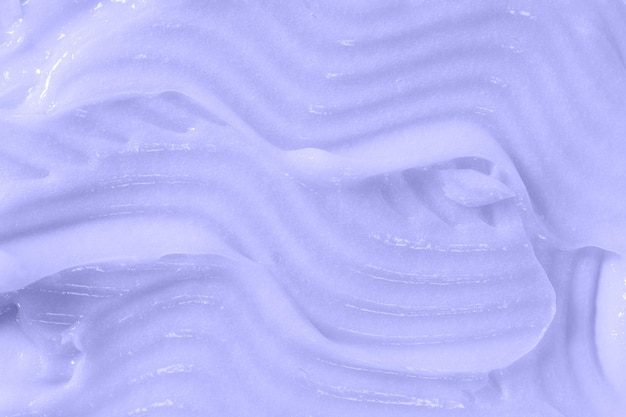This image features a close-up view of a creamy, viscous substance, portrayed in a horizontally rectangular format with no borders. The scene is dominated by various shades of blue, some so light they border on white, creating a harmonious background. Predominantly featured are intricate, wavy sections of a purple material, which appears to flow and exhibit a gel-like texture. The upper left corner of the image shows a slight shine as if light is reflecting off the surface. The substance seems to be arranged in three main segments with squiggly designs, possibly crafted with a serrated knife or similar tool. The design includes lines curving from the left to the upper right, right to the middle left, and another sweeping from the lower right, accentuating the fluid and textured nature of the material. The overall impression is of an artistic, yet indeterminate, silky gel or soap, presenting an enigmatic and tactile visual experience.